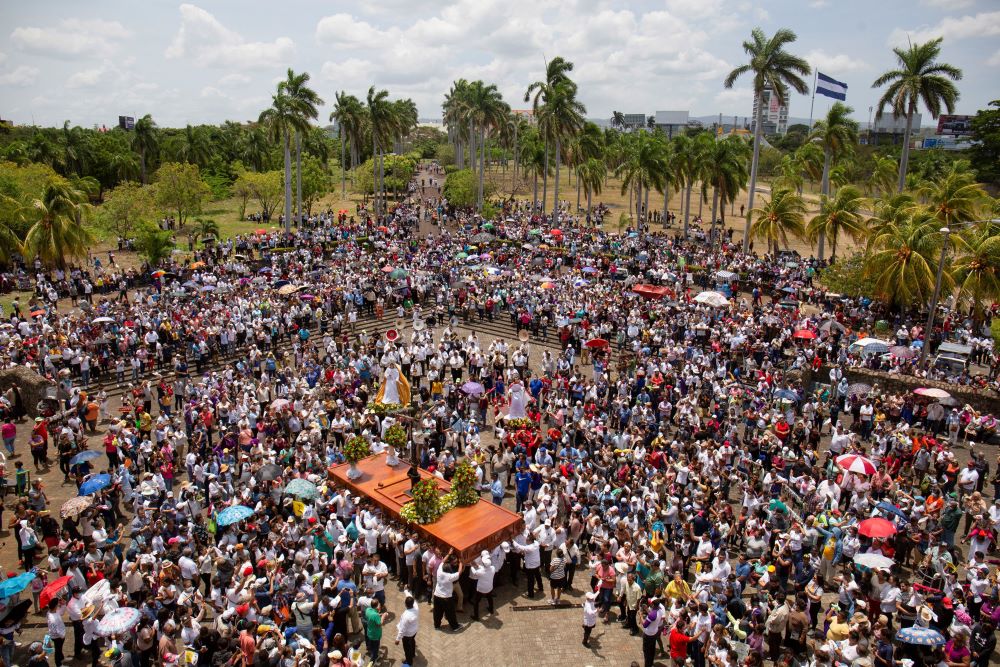This is a detailed, overhead color photograph captured by a drone, portraying a bustling outdoor event in a city center where a large crowd has gathered. The scene is filled with hundreds, if not thousands, of people, many of whom are holding umbrellas despite the cloudy weather. The crowd converges around a prominent wooden structure at the bottom center of the image, which resembles a stage or podium. This orange-colored podium, elevated above the crowd, is adorned with several floral arrangements and greenery. Atop this platform appears to be a cross with a figure of Jesus hanging on it, hinting at a religious aspect to the event.

Surrounding the main structure, people in white tops and black pants stand out, possibly participants in the event. Within the crowd, some individuals are holding musical instruments like trumpets. Stairs are visible in the upper part of the image, with people standing on them for a better vantage point. Farther back, additional figures can be seen on other platforms, wearing long robes that make them look like statues or officials.

Encircling the assembly, palm trees and an open field create a natural boundary. Additionally, a flag bearing blue and white stripes is positioned at the top right corner of the image, adding a touch of national or local significance to the gathering. The entire scene is set against a backdrop of representational realism, making the photograph a vivid capture of this large, organized event.